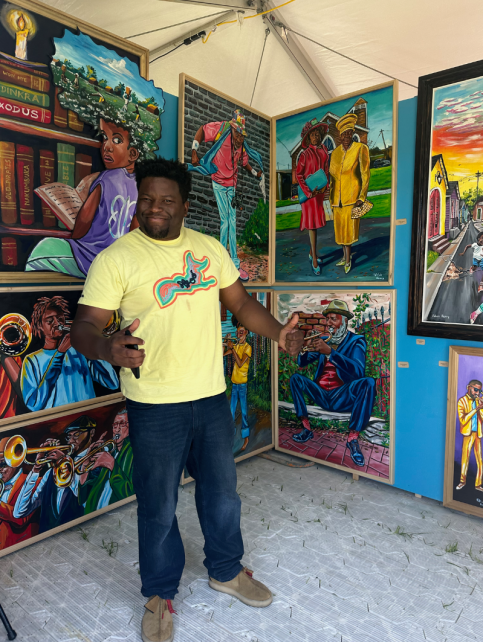In this vibrant photograph taken at an art fair or a small gallery, an African American man stands proudly amidst a richly-colored alcove of artwork, framed in thin wood frames, and displayed against an aqua blue wall. He is dressed in a yellow short-sleeve t-shirt with a design on the chest, blue jeans, and tan shoes. His short dark hair and closed-mouth smile radiate joy and pride as he gives a thumbs up. The white stone floor beneath him contrasts subtly with the vivid scenes in the paintings behind him, each depicting African American individuals.

To his left, there is a compelling painting of a black woman in a purple shirt and green pants, deeply immersed in a book in front of a towering bookcase. Below that, an energetic scene shows a black man in a long blue t-shirt playing the trumpet, accompanied by other musicians also playing trumpets. The lower right corner boasts a serene depiction of a man in a blue suit, seated on a low stone wall, playing a horn while wearing a tan hat. Meanwhile, the upper right corner illustrates two elegantly dressed women in bright yellow and red outfits, standing against a backdrop of a church and lush green grass, their attire complete with matching fancy hats and accessories. The artwork is filled with bright oil or acrylic colors and captures the cultural vibrancy and musical essence of the community.